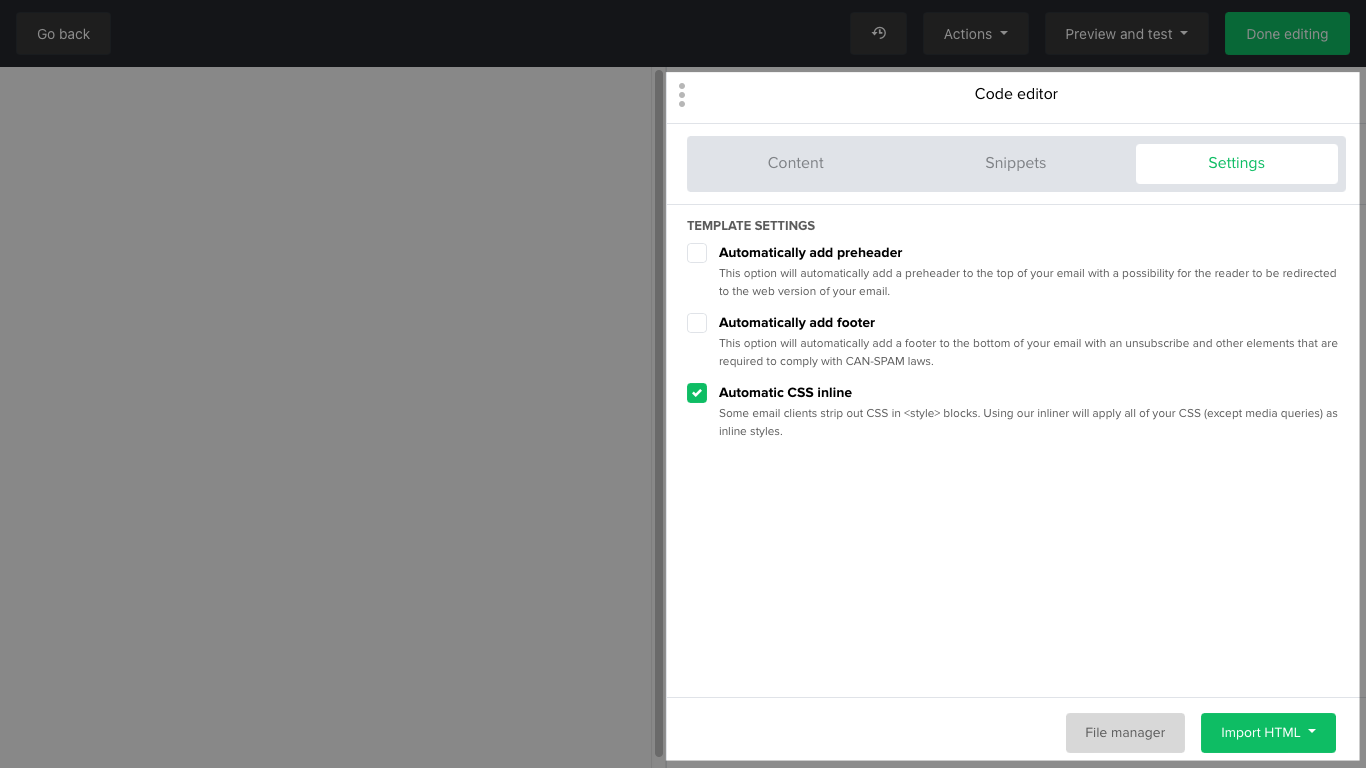The image depicts a computer screen in a landscape orientation. At the top, there is a black bar featuring several controls. On the left side of the bar, the text "Go Back" is visible, while the far right displays multiple options, including "Done Editing," "Preview and Test," "Actions," and a refresh button.

The main screen area is divided into two sections, with the smaller section on the right being completely empty and gray. The larger left section shows a code editor interface. This interface is set to display settings under tabs labeled "Consent," "Snippets," and "Settings," with "Settings" being currently active.

Within the "Settings" tab, several configuration options are listed, including "Template Settings," "Automatically Add Preheader," "Automatically Add Footer," and "Automatic Inline." The option "Automatic Inline" is selected, indicated by a tick mark. Unfortunately, some of the text appears too small to read clearly.